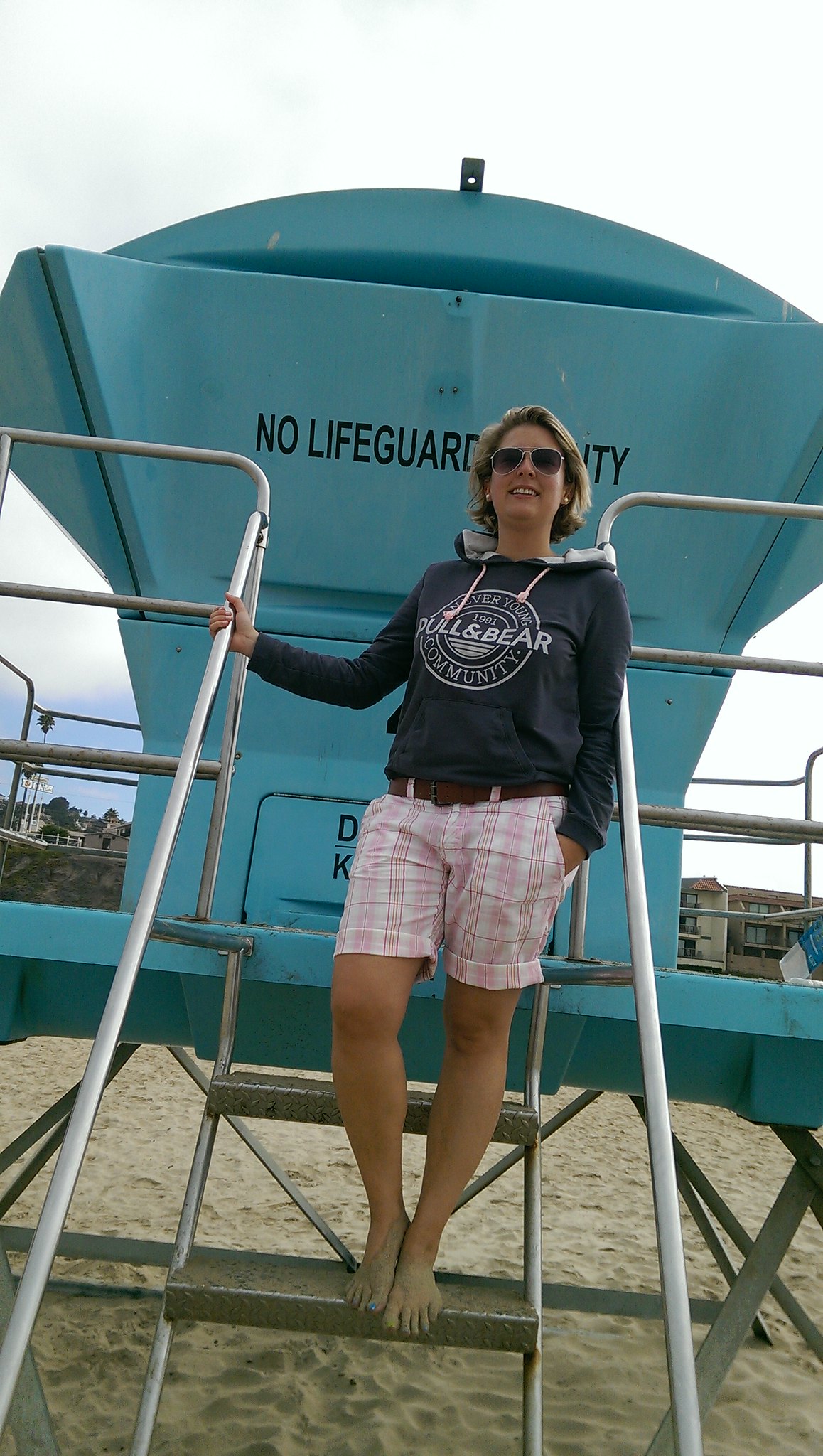On an overcast day at the beach, a woman stands on the metal steps of a unique, blue-green lifeguard stand with geometric shapes. The structure, topped with a round and triangular motif, bears a sign on the back reading "No lifeguard on duty," partially obscured by the woman. She has short blonde hair, wears dark sunglasses, and is dressed in a navy blue long-sleeve hoodie and white-and-red plaid shorts, suggesting an off-season setting. She stands barefoot, with one hand in her pocket and the other holding the rail. Surrounding her is trodden sand, and in the distance along the horizon, waterfront buildings and trees can be seen, adding to the serene, understated atmosphere of the scene.